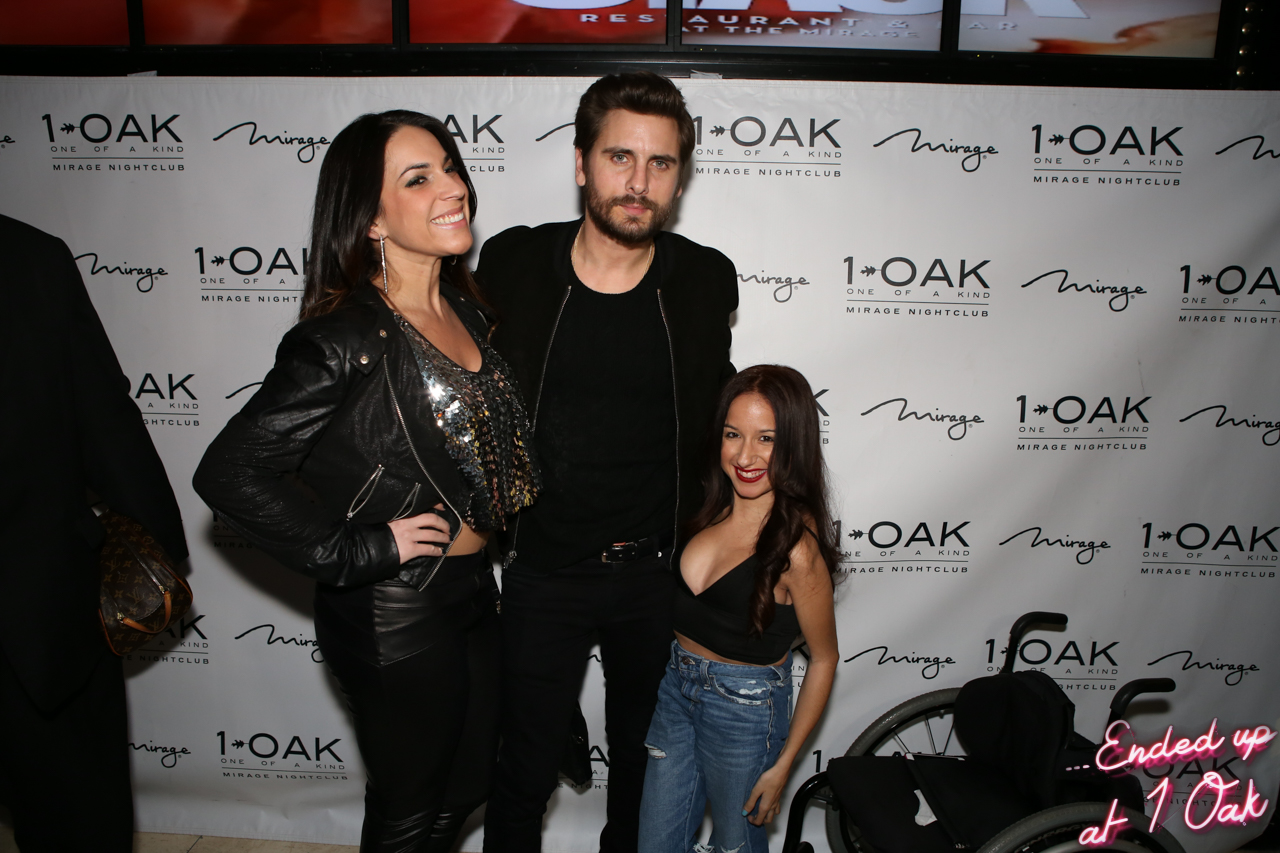In this photo taken at a nightclub, three individuals are posing in front of a step-and-repeat banner that reads "One Oak, One of a Kind, Mirage Nightclub." On the left is a woman with long dark hair, wearing a black leather biker's jacket, a silver sequined top, and dark pants. In the middle stands a man identified as Scott Disick, dressed entirely in black, including a black jacket, t-shirt, jeans, and a gold-buckled belt. His arm is around the woman to his left. On the right is a petite woman with brunette hair, dressed in a black halter top and denim jeans. A wheelchair is next to her. In the bottom right corner of the photo, neon pink cursive text reads, "Ended up at One Oak." Behind them, the backdrop features logos of One Oak and Mirage Nightclub.